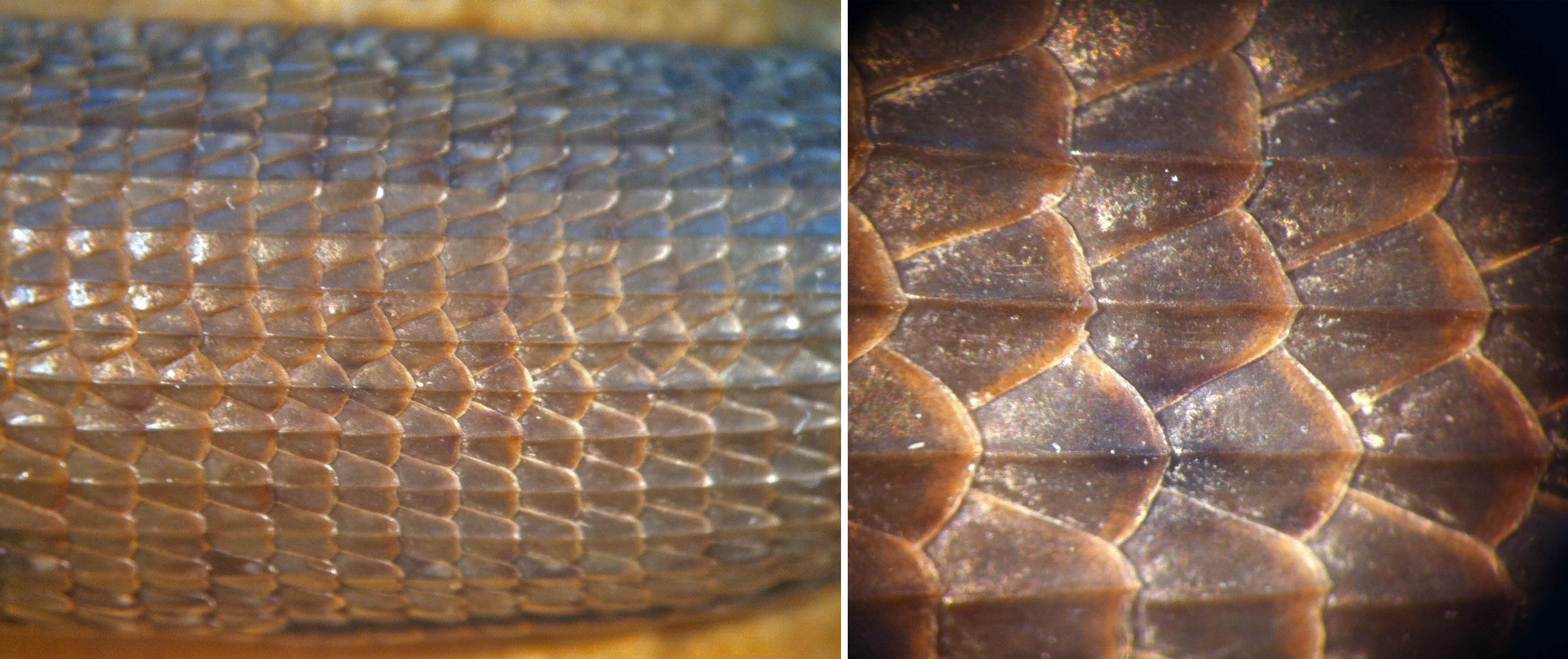This landscape-oriented image is divided into two vertical sections, showcasing a highly detailed close-up of what is likely snake skin. The left side displays a zoomed-out perspective featuring approximately 20 rows of interlaid brown scales. These scales, which span about three to four inches, exhibit a metallic sheen with varying hues of brown, lighter brown tips, and white flecks, giving a rusted, copper-like appearance. The upper rows carry a hint of bluish tint, while the lower rows transition to a darker brown. The very top and bottom edges of this section reveal a slight beige table background. The right side presents an even closer examination of the scales, highlighting their intricate, overlapping pattern. Here, the details become more pronounced, with the metallic, rusted effect more evident, and the scales displaying a mix of darker and lighter browns, along with blackish and gray tones accented by white specks. Both sections are framed by a subtle black border, focusing attention on the scaly texture that appears to shimmer under the light.